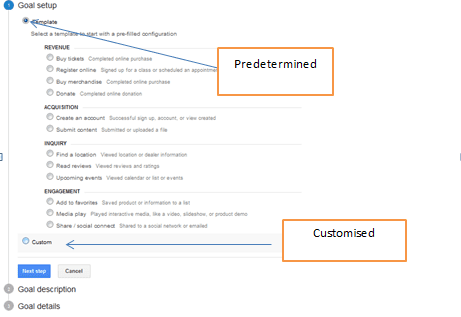**Webpage Snapshot Caption:**

This image captures a detailed view of a webpage with a clean white background. At the top, a thin grey line connects a series of circles. The first circle is blue with a white number '1' inside, labeled "Goal Setup" in bold black text. Following this blue circle are two dark grey circles, numbered '2' and '3', labeled "Goal Description" and "Goal Details" respectively, also in bold black text.

Below "Goal Setup," a highlighted bullet point with a blue dot indicates "This Template," situated next to bold text. A blue arrow extends from an orange-bordered box labeled "Predetermined" in bold black text, pointing toward the circle associated with "Goal Setup." Further to the right, another orange-bordered box labeled "Customized" in bold black points to a clickable button within a light grey rectangle labeled "Custom."

Underneath "This Template," a black text line reads "Select a template to start with a pre-filled configuration," followed by a bold black subheading, "Revenue." A series of clickable circles with varied tasks follow:

- "Buy Tickets"
- "Compare Online Purchase"
- "Regular Online" 
- "Signed Up for a Class or Schedule Appointment" (repeated twice)
- "Buy Merchandise" 
- "Completed Online Purchase" 
- "Donate" 
- "Complete Online Donation"

The next bold black subheading, "Acquisition," is followed by combined regular and bold black text entries: 

- "Create an Account"
- "Successfully Sign Up"
- "Account Review Created"
- "Submit Content"
- "Submitted or Uploaded a File"

The subsequent bold black subheading, "Inquiry," includes:

- "Find a Location"
- "Viewed Location or Daily Information"
- "Read Reviews"
- "Viewed Reviews and Ratings"
- "Upcoming Events"
- "Viewed Calendar or List of Events"

The final section, "Engagement," lists:

- "Add to Favorites"
- "Saved Product or Information to a List"
- "Media Play"
- "Played Interactive Media, like a Video, Slideshow, or Project Demo"
- "Share/Social Connect"
- "Share to a Social Network or Emailed"

This comprehensive layout elucidates the step-by-step process of goal setting and selection within the webpage interface, highlighting various options for revenue, acquisition, inquiry, and engagement.